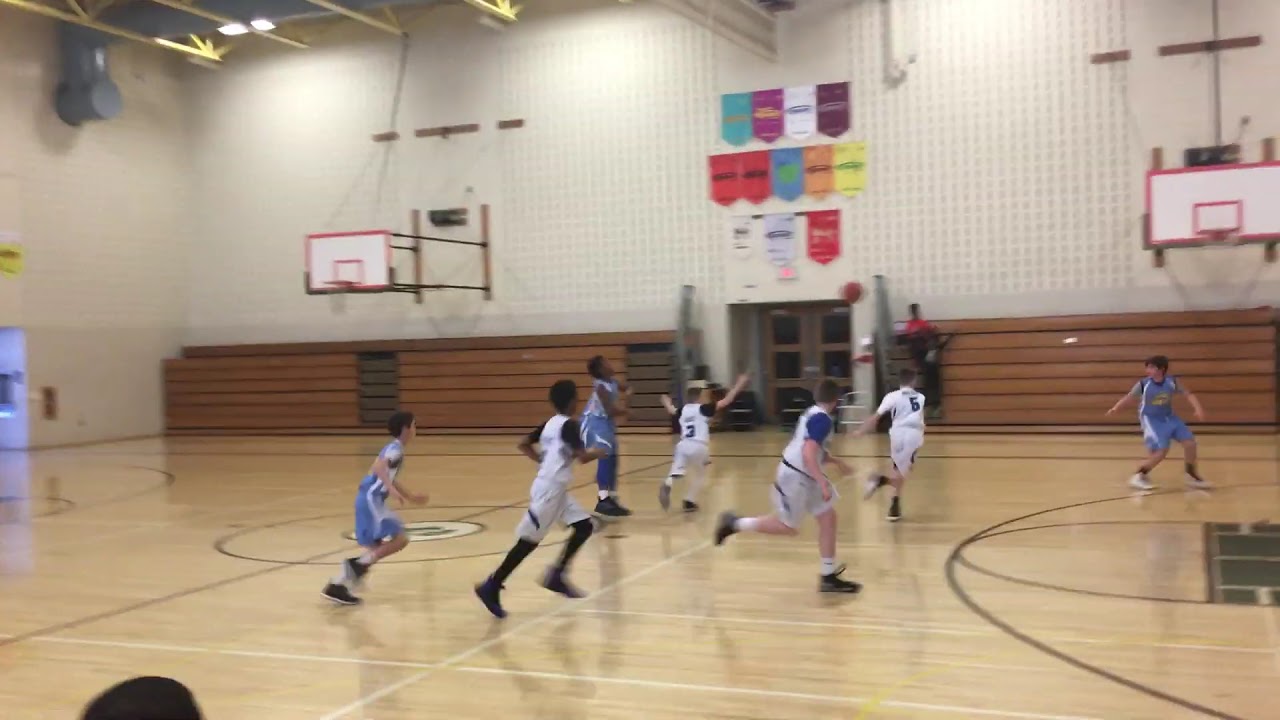The photograph captures an intense high school boys' basketball game taking place in an indoor stadium. The gym floor, a light brown hardwood, is prominently marked with white and black lines, leading to a central logo representing the home team. On the court, two teams are distinguishable by their uniforms: one team is clad in solid white with blue details, while the other sports solid blue with white details. Both teams are actively pursuing a red basketball, which is currently in mid-pass, underscoring the dynamic nature of the game. The background reveals brown bleachers pushed up against the wall, while above them colorful flags—blue, purple, white, green, and orange—hang on the upper part of the wall. The lower section of the wall is brown, transitioning to white above, and a door is situated in the middle, accented by various posters attached above it. Although no crowd is visible, the described scene emphasizes the players’ focus and the competitive atmosphere.